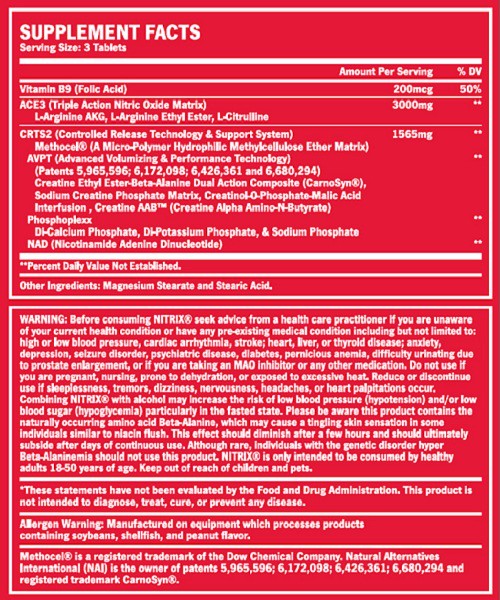The image is a detailed digital representation of a product label for Nitrix tablets, dominated by a red background with white text and outlines. At the top left, the label prominently displays "SUPPLEMENT FACTS" in all caps. Below this heading, it specifies a serving size of three tablets. A solid line separates this section from the listed supplement facts.

The tablet includes:
- **Vitamin B9 (Folic Acid):** 200 micrograms per serving, which constitutes 50% of the daily value.
- **ACE3:** 300 milligrams per serving (no daily value established).
- **CRTS2:** 1,565 milligrams per serving (no daily value established).

Following the ingredient details, it lists other ingredients such as magnesium stearate and stearic acid.

Underneath the supplement facts box, there is a prominent warning section advising users to consult a healthcare practitioner prior to use, particularly if they have pre-existing medical conditions like high or low blood pressure, cardiac arrhythmia, stroke, heart, liver, or thyroid disease, anxiety, depression, seizure disorder, psychiatric disease, diabetes, pernicious anemia, difficulty urinating due to prostate enlargement, or if they are taking an MAO inhibitor or any other medication. The warning also extends to nursing mothers advising not to take the supplement.

Furthermore, the label includes an allergen warning indicating that the product is manufactured on equipment that processes items containing soybeans, shellfish, and peanut flavor.

At the bottom, there are trademark details noting that Methadacil is a registered trademark of Dow Chemical Company, and National Alternatives International (NAI) is the owner of several patents mentioned. It also states that Carnosyn is a registered trademark. Additionally, it specifies that the statements have not been evaluated by the Food and Drug Administration, and the product is not intended to diagnose, treat, cure, or prevent any disease.